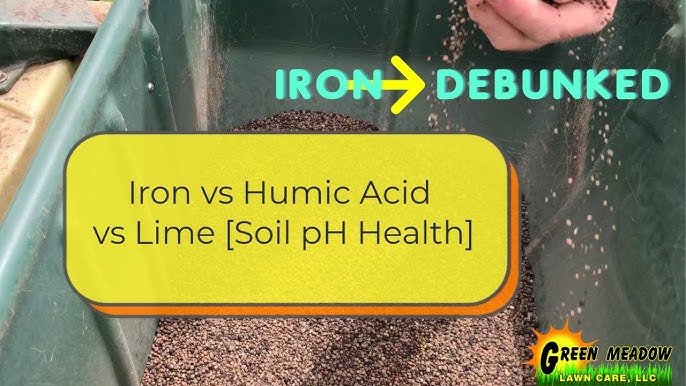The poster for Green Meadow Lawn Care Incorporated features a prominent header in blue text proclaiming "Iron Debunked" with an arrow connecting the words. Central to the poster is a large yellow box with black writing that reads "Iron vs. Humic Acid vs. Lime," and further clarifies in brackets, "Soil pH Health." In the background, an image depicts a hand releasing particles from a bin, possibly fertilizer or grass feed, allowing the substance to cascade down like rain. Additional bins are visible beside the main bin, though their contents remain unspecified. At the bottom right corner, the company name "Green Meadow Lawn Care Incorporated" is displayed, anchoring the poster's promotional message.